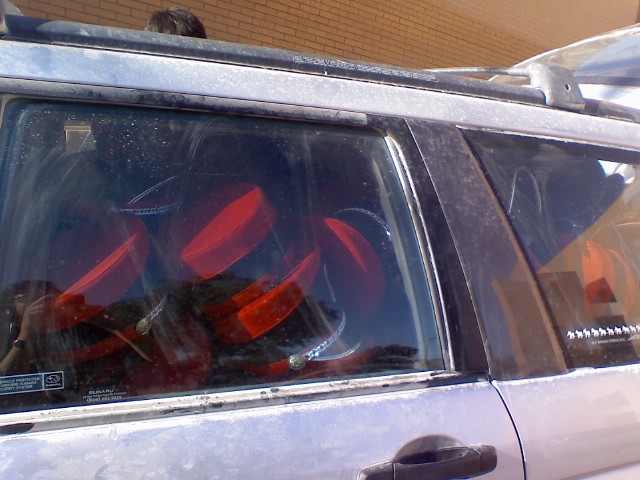This close-up photograph captures the side and partial rear of a silver estate car in poor condition, featuring prominent black trim including the door handles and roof rack. The image centers on the left rear door and the rear seat area, revealing several smudged and streaked windows through which an assortment of items can be seen. The windows are dirty with dried mud and partial smudges, indicating an attempt to wipe them clean. 

Inside the car, stacks of round, flat-topped red items are visible, with some reflective of hats, possibly costume or marching band headgear, though they could also be glass containers with red tops. These items are packed tightly both in the rear seats and the visible part of the boot, suggesting the car is filled with them. The car's trunk is slightly open, and more of these red items appear to be nestled inside. 

A light brown brick wall forms the background, and the top of someone's head is just visible over the roof of the car. In the bottom left corner, the reflection of the photographer, a lady wearing a watch, is seen in the car’s window, holding up a camera.